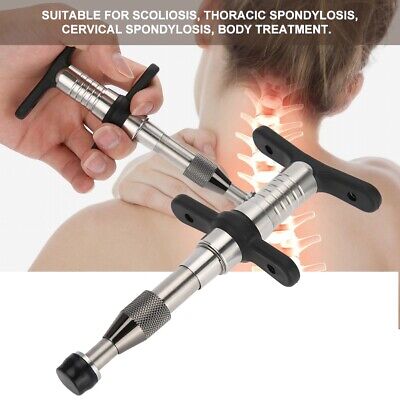The image is a medical advertisement for a device used in treating spinal issues such as scoliosis, thoracic spondylosis, cervical spondylosis, and for general body treatment. It prominently features a woman facing away, her hair pulled up to reveal the nape of her neck, and her right arm reaching across to her left shoulder. Superimposed on her back is a glowing outline of her spine, highlighting the spinal area. In the top left corner, another smaller image shows a person demonstrating the use of the device by holding it next to the woman's spinal cord, though it appears to be a staged example rather than an actual injection. The device itself, displayed prominently at the bottom of the image, is silver with black plastic components, including a plunger-like mechanism at its base. At the top of the image, white text reads, "Suitable for scoliosis, thoracic spondylosis, cervical spondylosis, body treatment."